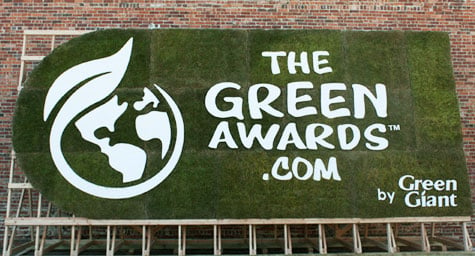This image features a large billboard-like sign, prominently displaying "thegreenawards.com" in bold, capitalized, white Sans Serif font. Positioned in the bottom right corner is the text "by Green Giant." The sign has a unique design, combining a rectangular shape on the right with a rounded, circular edge on the left, allowing a glimpse of the metal scaffolding that supports it. A globe with a leaf extending from the top is centrally featured, symbolizing environmental consciousness. The overall color scheme is dominated by a rich, dark green background contrasted by the white font and globe. The sign appears to be mounted on a tan metal stand, positioned outside against a brick wall, with no visible shadows, suggesting it was taken in good lighting conditions.